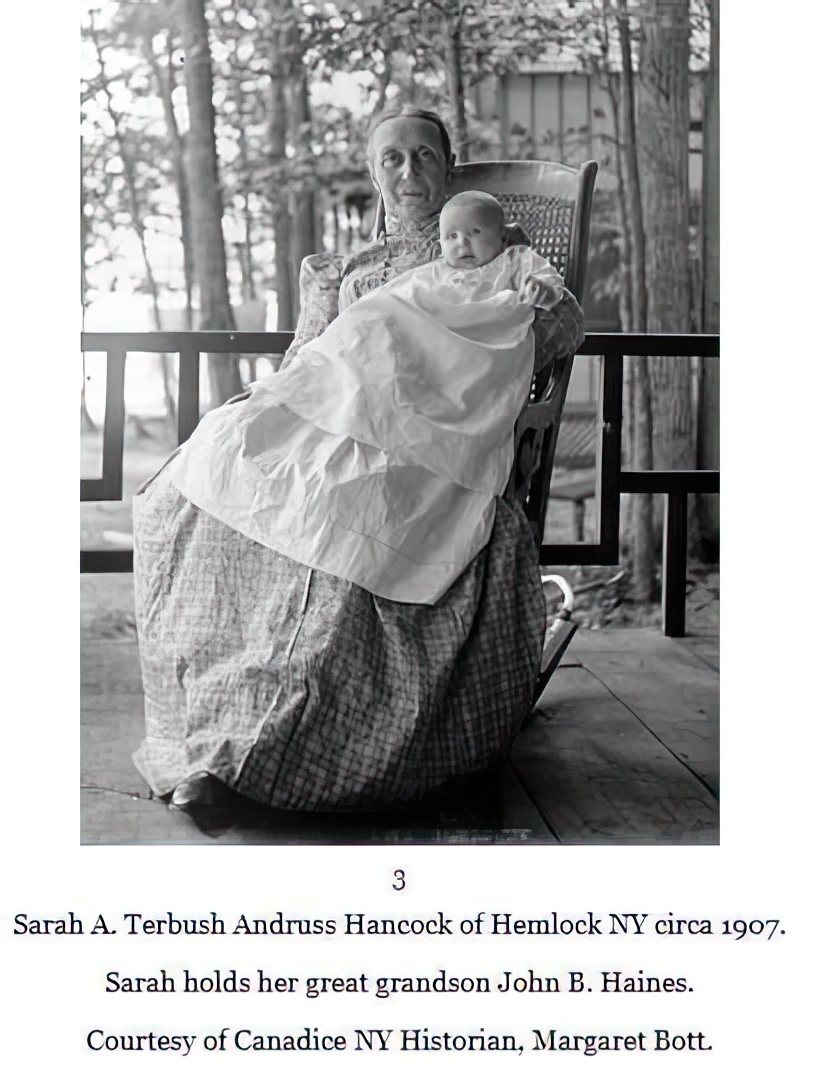This black and white photograph, taken circa 1907, captures an elderly woman, identified as Sarah A. Turbush Andras Haak Hancock of Hemlock, New York, seated in a wooden rocking chair on an old wooden porch. She is holding her under-one-year-old great-grandson, John B. Haynes, who is dressed in a remarkably long white robe. Sarah, likely in her 80s, is wearing a long, checkerboard-patterned dress with poofy sleeves and a voluminous skirt. Both are facing the camera, Sarah with a somewhat challenging attempt at a smile due to her age, and the baby gazing directly ahead with barely open eyes. The porch features geometric, squared railings, and the background reveals a dark-colored fence, trees, and another building with vertical slats, suggesting a daytime setting. The photograph, remastered for historical preservation, is accompanied by text attributing the image to Candace, New York historian Margot Bott.